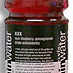The image depicts a very small, blurry picture of a bottle of Vitamin Water. The bottle is clear, containing a purplish-red liquid, hinting at a berry or possibly dragon fruit flavor. The label of the bottle is black and white, with the word "Vitamin" partially visible and "Water" legible on each side of the label. Although the text on the label is mostly unreadable due to the image's low resolution and pixelation, the main colors identifiable in the picture are red, black, and white. The image is so blurry that without previous knowledge of what Vitamin Water bottles look like, it would be challenging to recognize. The background of the image is predominantly white, but it's barely noticeable as the bottle image takes up most of the frame.